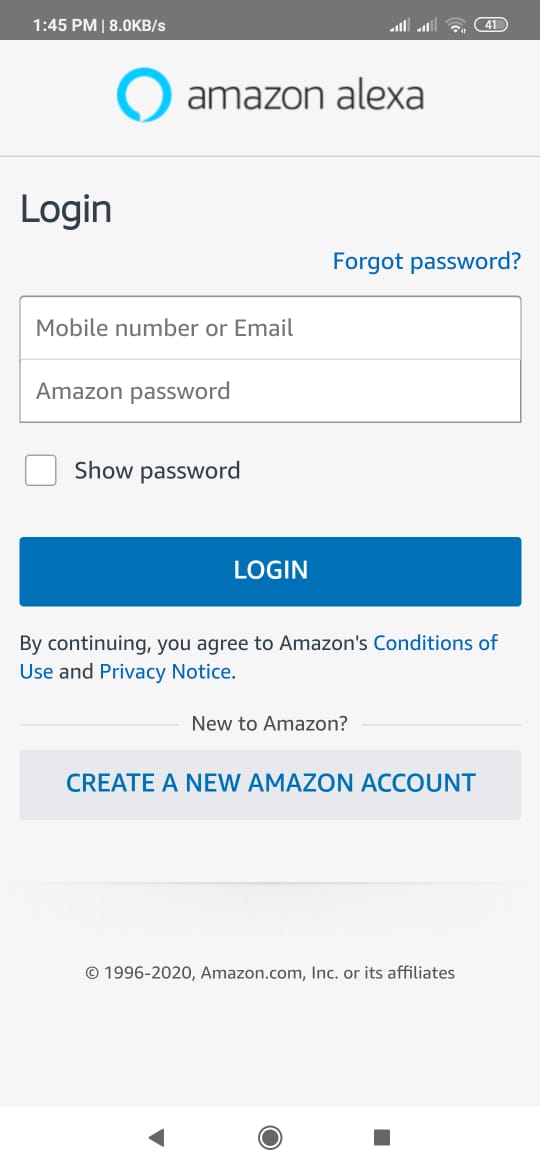**Detailed Caption:**

The image is a screenshot from a website interface with several distinguishable sections and elements.

- **Header Section:**
  - A dark charcoal gray banner at the top displays the current time "1.45 p.m." in white text.
  - Adjacent to the time, a vertical line separates it from the data indicator "8.0 KB/s" where "KB" are capitalized, and "s" is lowercase.
  - On the right side of this banner, icons for two cell signals, a Wi-Fi signal, and a battery symbol with "41%" charge are visible.

- **Main Interface:**
  - The background below the banner is a lighter gray.
  - Positioned towards the left, a vibrant bright ocean blue circle features prominently.
  - Next to the blue circle, "Amazon Alexa" is written in lowercase white text.

- **Login Section:**
  - Below this, a horizontal line separates the Amazon Alexa title from the login section.
  - On the left, "Login" is indicated in capital "L" and black text, while to the right, "Forgot password?" is displayed in blue text with a capital "F" and a question mark at the end.
  - Further down, there is a distinct rectangle divided into two fields:
    - The top field prompts for "Mobile number or email," with capital "M" in Mobile and capital "E" in Email.
    - The bottom field requests the "Amazon password", capitalizing the "A" in Amazon and the "P" in Password.

- **Additional Options:**
  - Outside of the input fields, a small white square with a gray trim offers the option to "Show password," with a capital "S".
  - Underneath, a blue banner labeled "Login" in white text stands out.
  - Text below the login button reads: "By continuing, you agree to Amazon's Conditions of Use and Privacy Notice."
  - A final notice encourages new users with the message, "New to Amazon? Create a new Amazon account."

This detailed description provides a comprehensive overview of the website's screenshot, clearly outlining all visible elements and text.